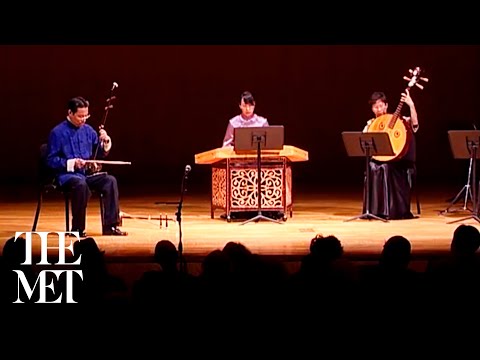In this captivating image from an indoor concert at The Met, three skilled musicians are illuminated under a single, bright spotlight against a backdrop of darkness. The concert hall is filled with a captivated audience, visible only by the silent silhouettes of their heads. The stage, a light-colored wooden platform, hosts the performers who appear to be engaging with traditional Asian musical instruments.

On the left, a gentleman in a bright blue traditional Asian tunic with white cuffs, dark pants, and glasses, sits with a fiddle-like instrument held in his lap, using a bow with his right hand. The center spot is occupied by a lady with dark hair, playing a large lap harp positioned in front of her on a stand, with sheet music carefully arranged ahead of her. To her right, another woman, dressed in a long black skirt, expertly handles a large, round-bodied string instrument with a long neck, identifiable by its four tuning pegs. This performer, too, is accompanied by a sheet music stand in front of her.

Further to the right, a final stand presides with no visible performer, accentuating the serene blackness that envelops the background of the stage. The elegant simplicity of "The Met" logo, placed in large white letters, subtly marks the lower corner of this timeless and evocative performance.